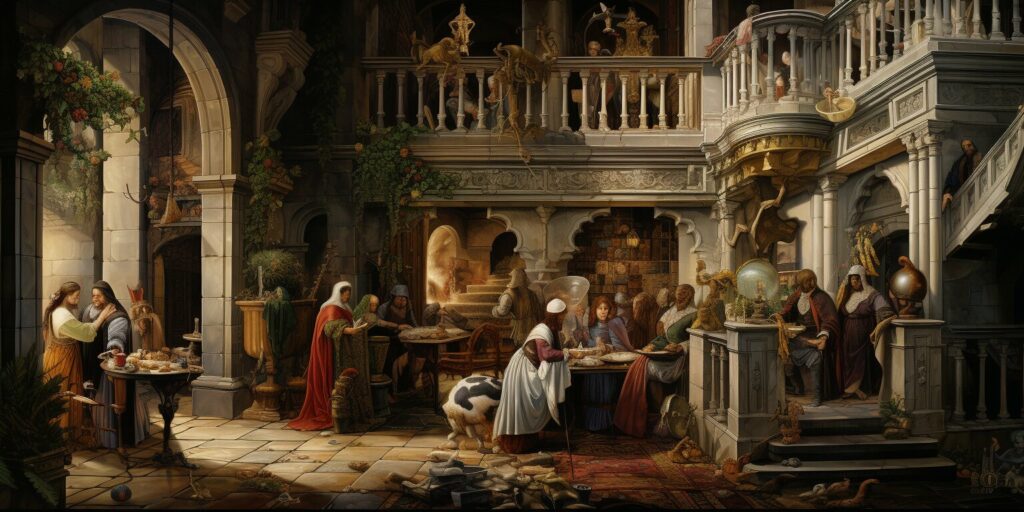This masterfully detailed Renaissance painting captures a lavish get-together in what appears to be a grand, two-story monastery. The complex architecture, adorned with ornate gold accents and vibrant blue hues, suggests a setting fit for nobility. People dressed in colorful robes of red, brown, blue, and black mingle in an intricate scene. The lower level of the building features tables laden with bread and wine, and the animated crowd is immersed in conversation and communal activities. Some women in the background seem to be preparing food, while others stand or sit around the tables. The upper story, with its decorative sculptures and a gated balcony, appears less populated but may have hidden figures. Light pours in from the left through stone pillars, illuminating a courtyard where animals and bales of hay are visible. This diverse, bustling composition, marked by its rich colors and detailed interactions, underlines the artist's mastery and the timeless elegance of the Renaissance period.